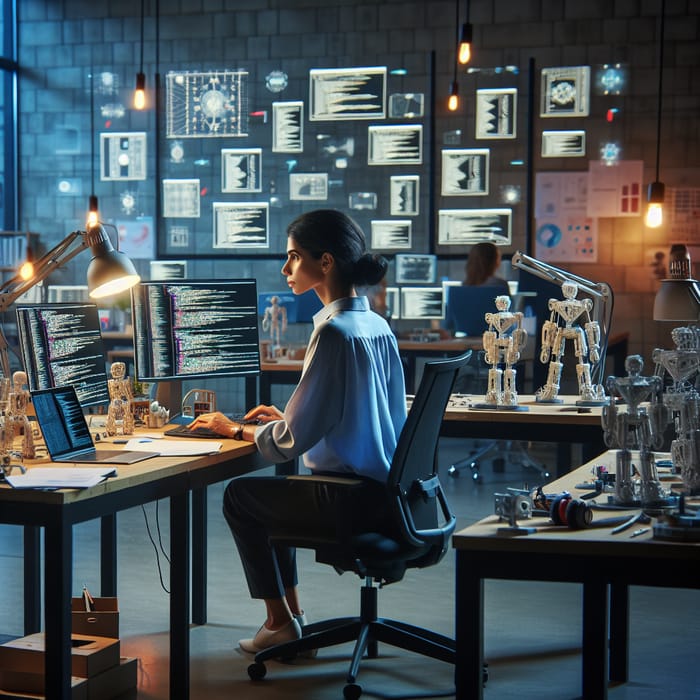This detailed, computer-generated 3D rendered image portrays a realistic yet slightly cartoonish office setting. In the foreground, a focused woman with her hair tied in a bun sits in an office chair at the center. She is dressed in a blue collared shirt and jeans, finishing off her look with shoes. In front of her, she has three computer screens—one from a laptop and two desktop monitors—all displaying indecipherable code. Surrounding her, the workspace is cluttered with small robotic models, some placed on tables to her right and appearing to be 3D printed.

The back wall of the office is a textured brick wall adorned with projected screens and posters, which feature running code, models, and scientific graphs. Another co-worker, also engrossed in her work, is situated against this wall, working at her desk equipped with multiple monitors. Various lamps and office fixtures add to the high-tech, meticulous ambiance of this workspace.